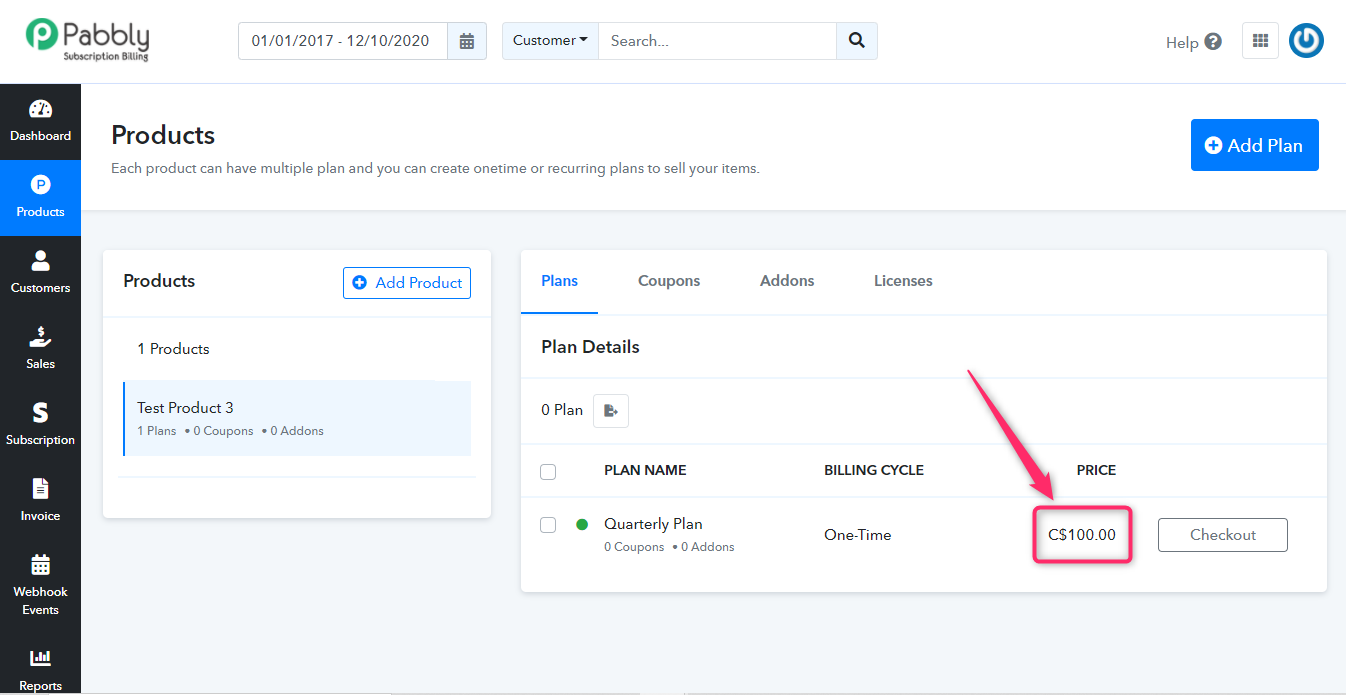This screenshot captures the Pabbly Subscription Billing interface in detail. At the top-left corner, the Pabbly logo is prominently displayed, represented by a green icon with a white "P." Adjacent to the logo, the date range from January 1st, 2017, to December 10th, 2020, is selectable with a small calendar icon for date adjustment. A search bar labeled "Customer" is also visible for user convenience. On the top-right, there are several utility icons: a help icon denoted by a question mark, a nine-block menu icon for additional options, and what appears to be a refresh icon.

The vertical black sidebar on the left-hand side of the screen hosts multiple navigational icons. The dashboard icon is prominently positioned at the top. Below it, the "Products" section is highlighted in blue, followed by sections for "Customers," "Sales," "Subscription," "Invoice," "Webhook," "Events," and "Reports."

In the central part of the interface, the top header reads "Products." Below this heading is a description explaining that each product can have multiple plans, including one-time or recurring plans. To the right, a blue rectangular button labeled "Add Plan" is available for creating new plans. 

Beneath this, a white box lists existing products. For instance, "Test Product Three" is displayed with details indicating one plan, zero coupons, three somethings, and zero add-ons, along with an option to add more products.

To the right of this list is a larger white rectangular box featuring various options such as "Plans," "Coupons," "Add-Ons," and "Licenses." Detailed plan information is provided within this section, including the "Plan Name" labeled "Quarterly Plan," its "Billing Cycle" set to "One Time," the price listed as Canadian $100, and a "Checkout" option for purchasing plans.